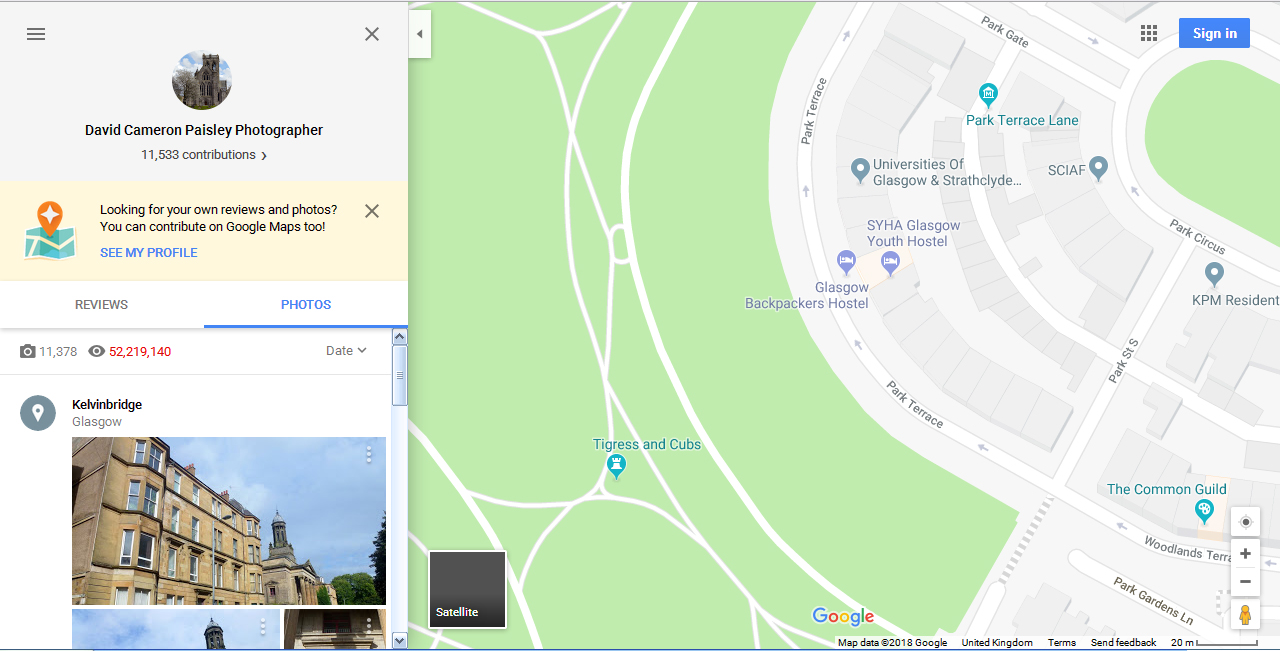This image is a detailed screenshot taken from Google Maps. Dominating the right side, which takes up about 65-75% of the screen, is a map showcasing a specific area in Glasgow, including locations like Glasgow Backpackers Hostel, SYHA Glasgow Youth Hostel, the Common Guild, and Park Terrace. The map reveals street names, white road lines, and green spaces where there are no roads. On the left side, there are two notable sections: the top half displays the business name, "David Cameron Paisley Photography, Photographer," indicating the photographer's profile and contributions. Directly below, the bottom half of the left side shows images related to the business, specifically photos of the Kelvin Bridge in Glasgow. Additionally, a sign-in button is visible in the top right corner, suggesting the screenshot was taken from a computer, with the Google logo also visible at the bottom middle of the image.